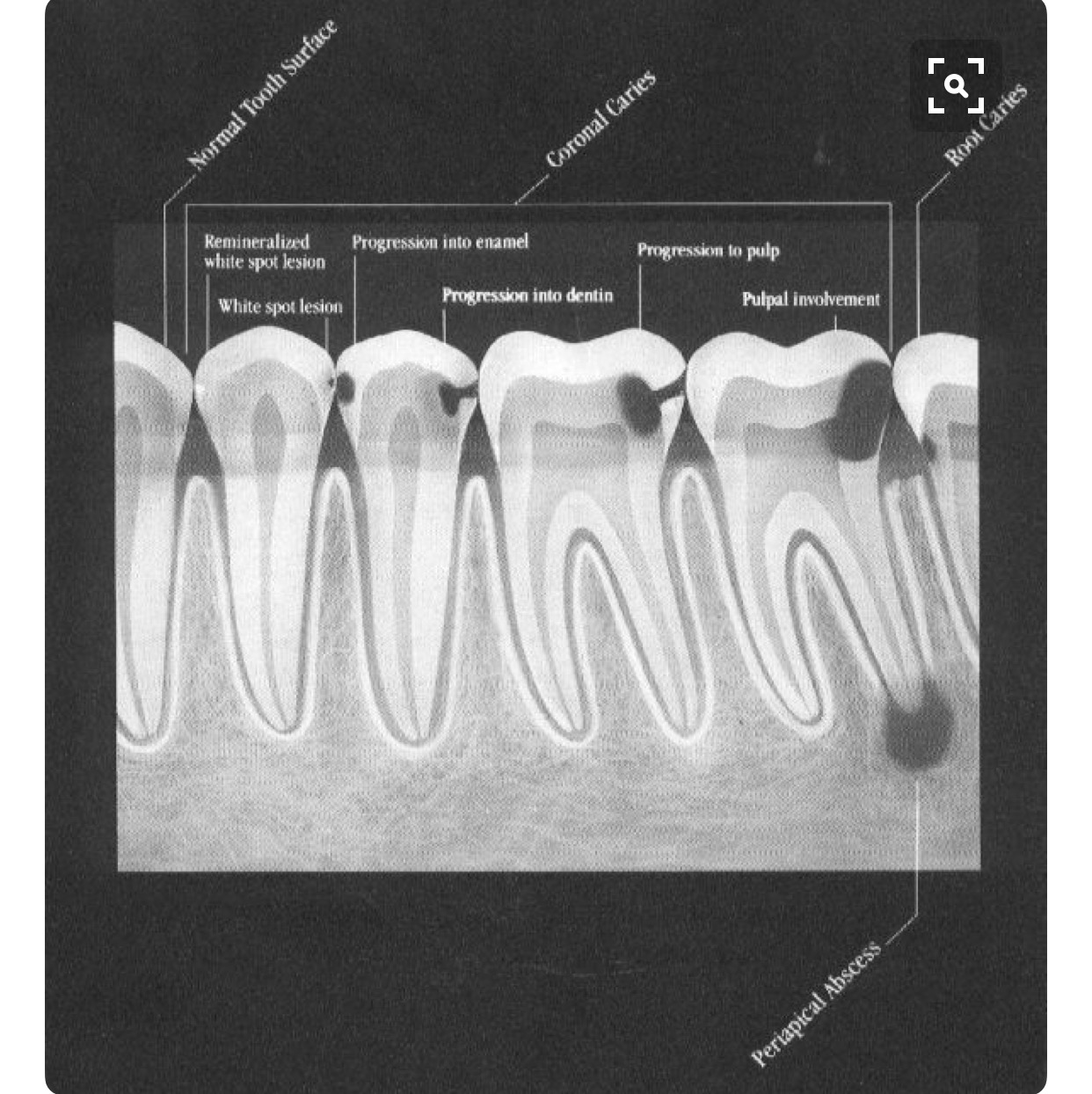This image features an artist’s detailed sketch of a dental x-ray set against a stark black background. Centered within the frame is a depiction of teeth, including molars and premolars, with precise labeling. The teeth are highlighted in white, illustrating various stages of dental conditions. The text across the top sequentially labels these conditions from left to right as "normal tooth surface," "remineralized white spot lesion," "white spot lesion," "progression into enamel," "coronal caries," "progression into dentin," "progression into pulp," "pulpal involvement," "root caries," and "periapical abscess." The x-ray-like drawing shows both the crown and roots of the teeth, along with the gum line depicted in a whitish-gray hue. In the upper right-hand corner, a small icon resembling a transparent square with white bracket-like triangles and a magnifying glass subtly invites a closer inspection. This diagram meticulously points out different stages and maladies associated with the teeth.